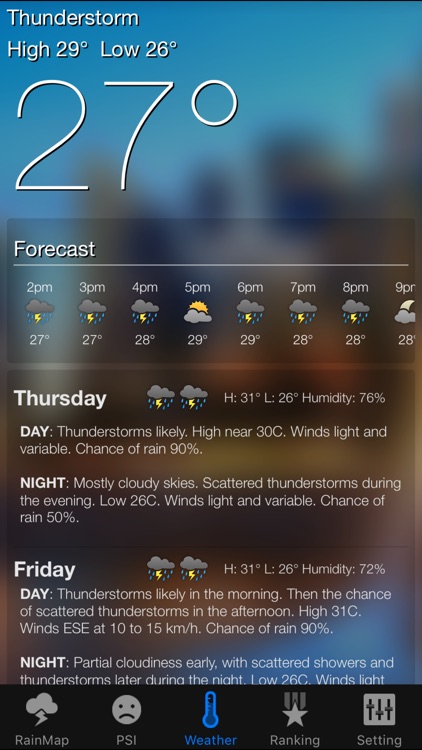Current weather conditions are characterized by thunderstorms and moderate temperatures. At 3 p.m., the temperature is 27°C, rising to 28°C by 4 p.m., and peaking at 29°C by 5 p.m. when there is a mix of sun and clouds. The temperature remains steady at 29°C at 6 p.m., then slightly decreases to 28°C from 7 p.m. through 9 p.m., with the later part of the evening showing a cloudy sky with a moon icon.

**Thursday's Forecast:**
- **Day:** Thunderstorms are likely, with temperatures reaching a high of 31°C and a low of 26°C. Humidity is at 76%, with light and variable winds. The chance of rain is 90%.
- **Night:** The skies will be mostly cloudy, with scattered thunderstorms possible during the evening. The low will remain at 26°C, with light and variable winds, and a 50% chance of rain.

**Friday's Forecast:**
- **Day:** Expect cloud cover with thunderstorms, similar to the previous day. The high will be 31°C and the low 26°C, with a humidity level of 72%.